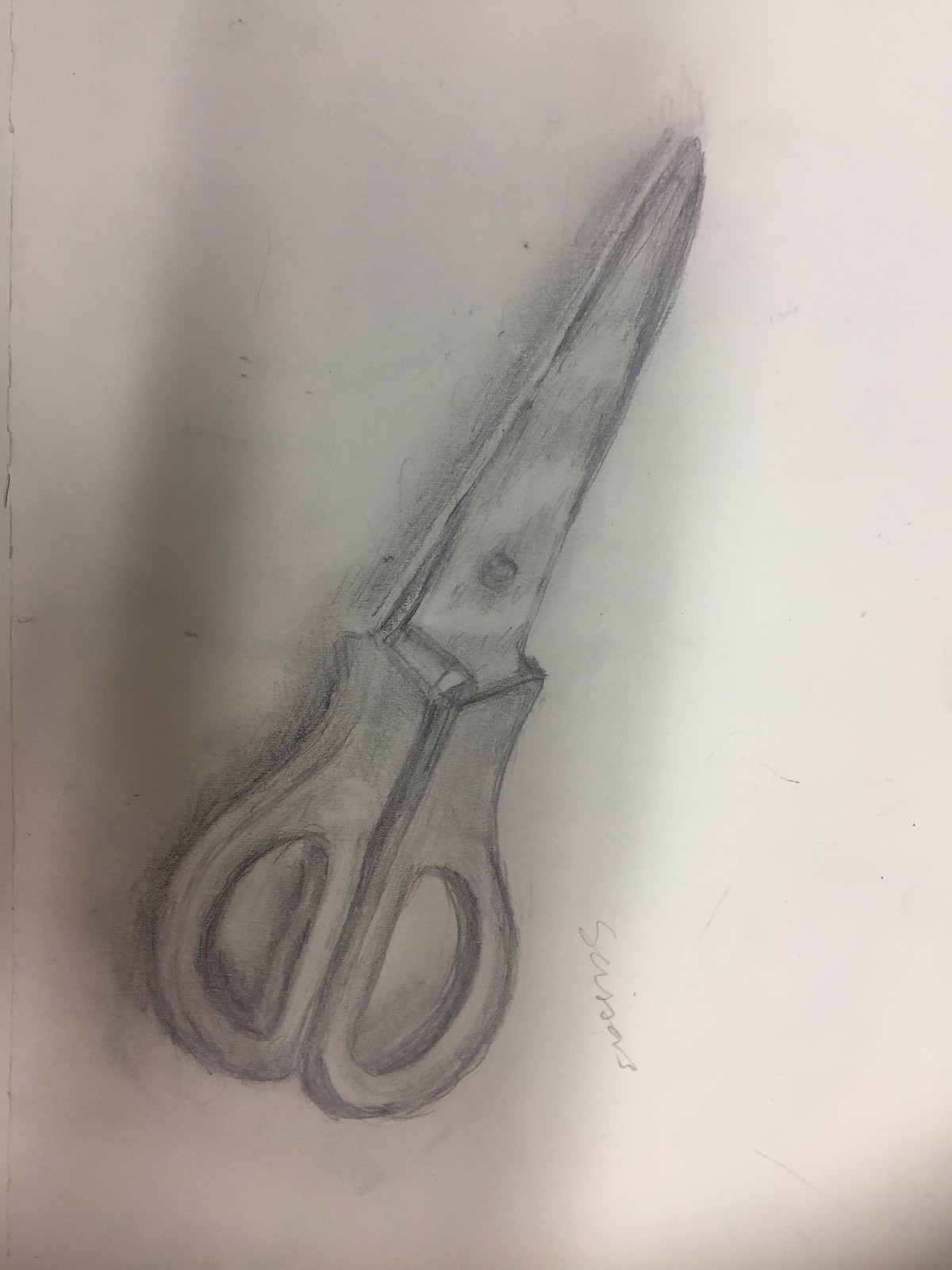This detailed pencil sketch depicts a pair of closed scissors with precision and artistry. The scissors feature large, oval-shaped finger holes designed for comfortable handling. The handles are rendered in plastic, juxtaposed with blades that exhibit meticulous shading to evoke a metallic sheen, adding a realistic touch to the drawing. The word "scissors" is inscribed in elegant cursive along the side, enhancing the overall authenticity and intricacy of the artwork.